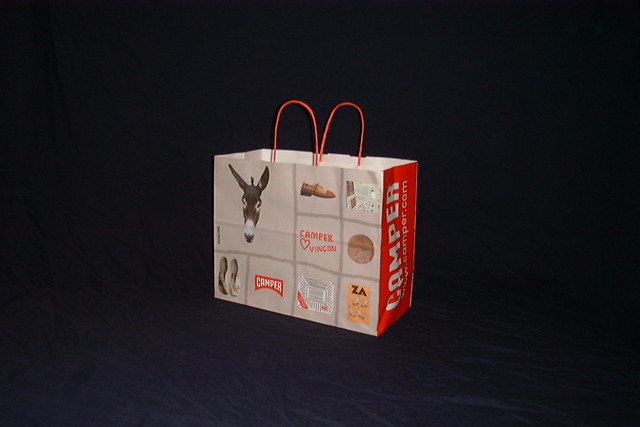This image depicts a single gray paper shopping bag set against a pitch-black background with subtle texture, possibly indicating a navy blue or dark gray surface. The shopping bag is detailed with various elements and designs. Prominently, it features two thin red handles on either side. The bag bears the Camper brand name in white letters on a red side panel, along with the website "www.camper.com." The front of the bag is divided into a series of squares of different sizes, each showcasing distinct images and text. One square displays a brown donkey head with a white nose, another shows a pair of brown shoes, while yet another features slip-on type shoes. There's also the repeated Camper Vincon logo with a heart. The composite elements give the appearance of a meticulously crafted piece of artwork, blending the brand's logo, product images, and decorative motifs.